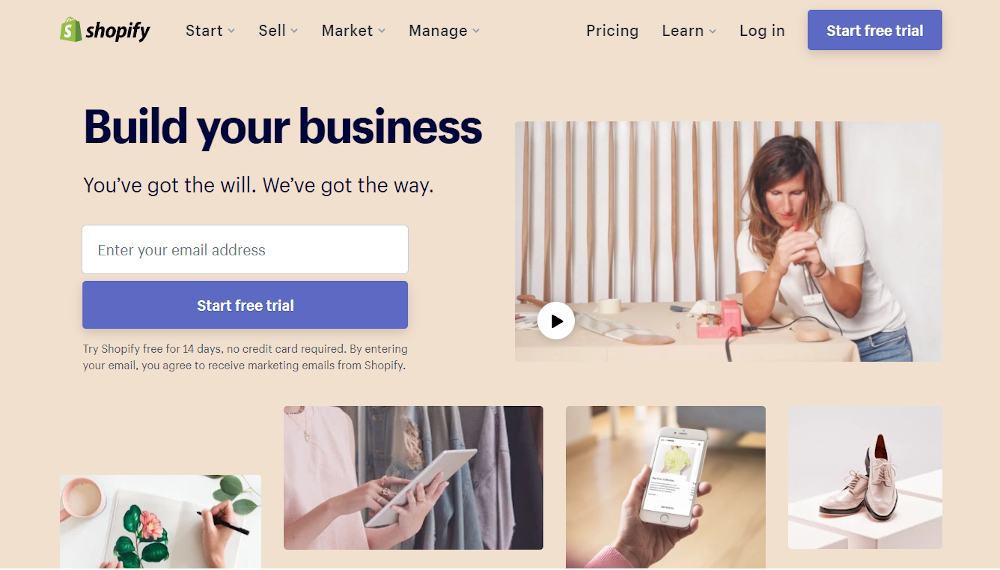A screenshot from the Shopify website is displayed, prominently featuring the tagline, "Build your business. You've got the will, we've got the way." Below this, there's a prompt to enter your email address and a "Start Free Trial" button. The website's header boasts the Shopify logo—a shopping bag with an "S" on it—and navigation tabs labeled Start, Sell, Market, Manage, Pricing, Learn, Login, and Start Free Trial. The screen also includes a small video icon for a playable clip. Scattered across the page are various images: one showing someone drawing a flower on a piece of paper, another of a person using a tablet, yet another of someone holding a smartphone, and an image of shoes displayed on a table, hinting at the types of products users can sell on the platform.